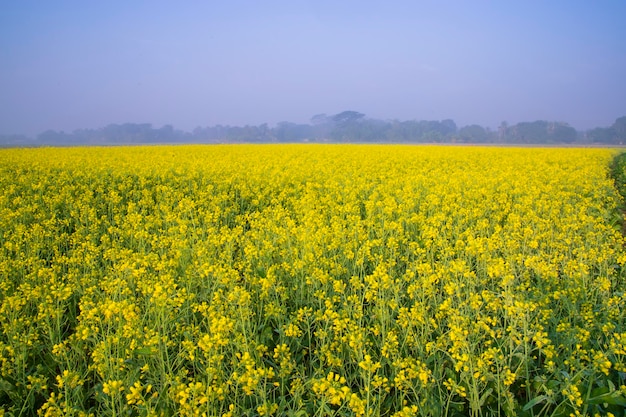This photograph captures a vast, flat field covered in yellow flowers, extending as far as the horizon. In the foreground, green leaves and long stems are visible, supporting the vibrant yellow blooms, which become denser as the view extends further into the distance. The field appears almost solid green due to the abundance of foliage. At the distant horizon, a line of vague, bluish-gray trees marks the boundary of the field, while the hazy, purplish-blue sky above adds a dreamy quality to the scene. To the left side of the image, a bush slightly protrudes into the yellow expanse, and a small shrub appears halfway along the right edge. There are also some indistinct buildings visible at the horizon, and the flowers, potentially of an edible variety, seem to be awaiting harvest.